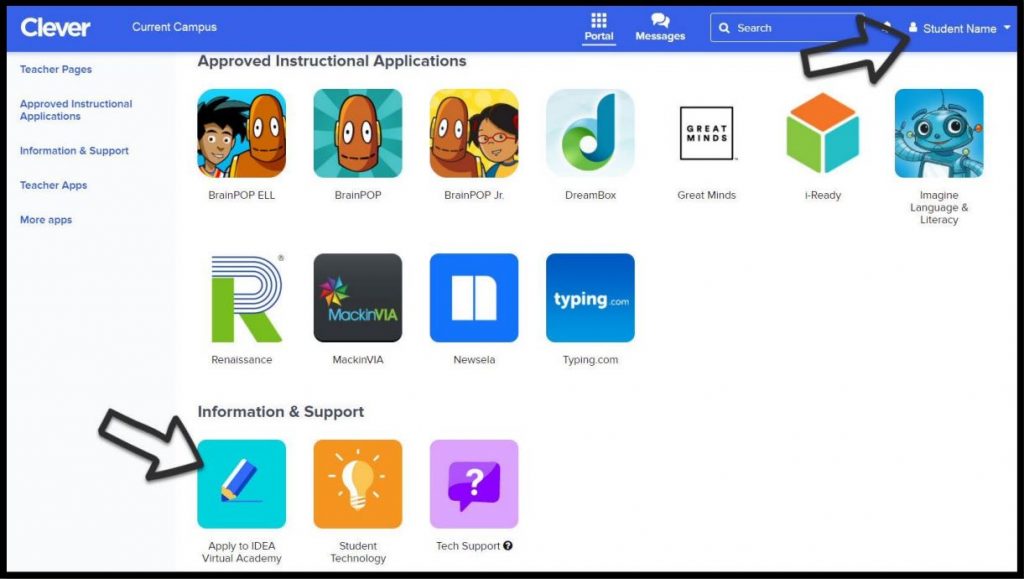The image displays the Clever app interface, prominently featuring a blue rectangular header with the word "Clever" in white text, followed by "Current Campus." Below this, "Portal" is displayed alongside an icon consisting of nine small squares, denoting that this section is currently selected. Adjacent to this, the "Messages" section is identified by two speech bubble icons. Further down, there is a search bar equipped with a magnifying glass icon for user queries, a notification bell icon, and a profile picture area labeled "Student Name" accompanied by a drop-down triangle.

The image has been annotated with a large black arrow pointing towards the "Student Name" section. Another arrow, located at the bottom of the image, will be discussed subsequently. On the left side of the interface, a side menu lists various sections: "Teacher Pages," "Approved Instructional Applications," "Information and Support," "Teacher Apps," and "More Apps."

Within the "Approved Instructional Applications" section, several educational tools are displayed, including:

- BrainPOP ELL
- BrainPOP
- BrainPOP Jr.
- DreamBox
- Great Minds
- iReady
- Imagine Language and Literacy
- Renaissance
- MacinVIA
- NewsELA
- Typing.com

Each application is represented by distinct thumbnails, such as DreamBox's blue and green "D," and iReady's 3D box with blue, orange, and green sides. Typing.com is noted with a blue rectangle bearing the site's name in white text.

An additional annotation points to the "Apply to IDEA Virtual Academy" option within the "Information and Support" section. Adjacent to it, "Student Technology" and "Tech Support" (shown with a white question mark inside a black circle) are also visible. This detailed interface representation demonstrates how users can navigate to their student profile and apply to the IDEA Virtual Academy.